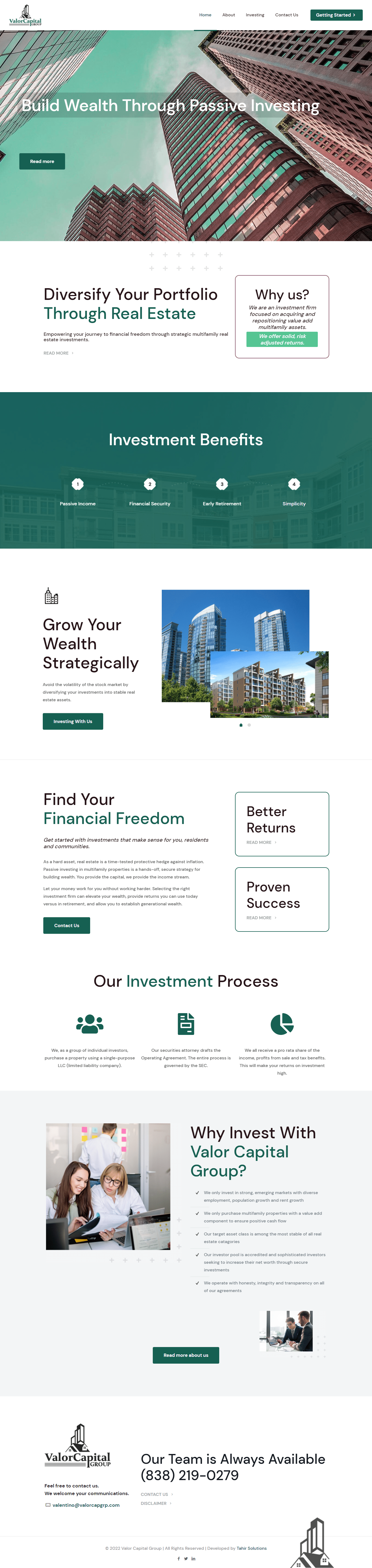This image was taken from a website but is extremely blurry, making it difficult to discern the specific content. The dominant theme color appears to be a mixture of green and teal, which is used in various shades throughout different text boxes and sections. At the top of the image, there's a photo showcasing a cityscape with a viewpoint directed upwards towards three high-rise buildings. Unfortunately, the text at the top of the image is unreadable due to the blurriness.

Below the main image, there is some text that is partially legible, which seems to suggest diversifying your portfolio through real estate. Further down, there is a darker, deep-sea green text box, possibly highlighting the benefits of some kind of studio service. This section is followed by four icons that presumably represent various benefits offered by the website.

The next section contains beneficial points organized into two paragraphs on the left-hand side, accompanied by an image. Below this are two text boxes on the right-hand side. Here, there are two images of different buildings against a blue sky, further emphasizing the real estate theme. A text area beneath these images might mention some sort of process, accompanied by three icons indicating integration with other services or connections.

Towards the bottom of the image, there is a photograph of two people looking down at what could be an iPad or a book. One is a younger woman with long hair, and beside her is an older woman with short hair and glasses. In the background, a man is walking away from the camera. The women are wearing white, while the younger woman may be dressed in a gray shirt. Adjacent to this image, there is text possibly related to the reasons for connecting or investing with a certain capital group, though the exact name remains unclear—perhaps something akin to Faker Capital Group.